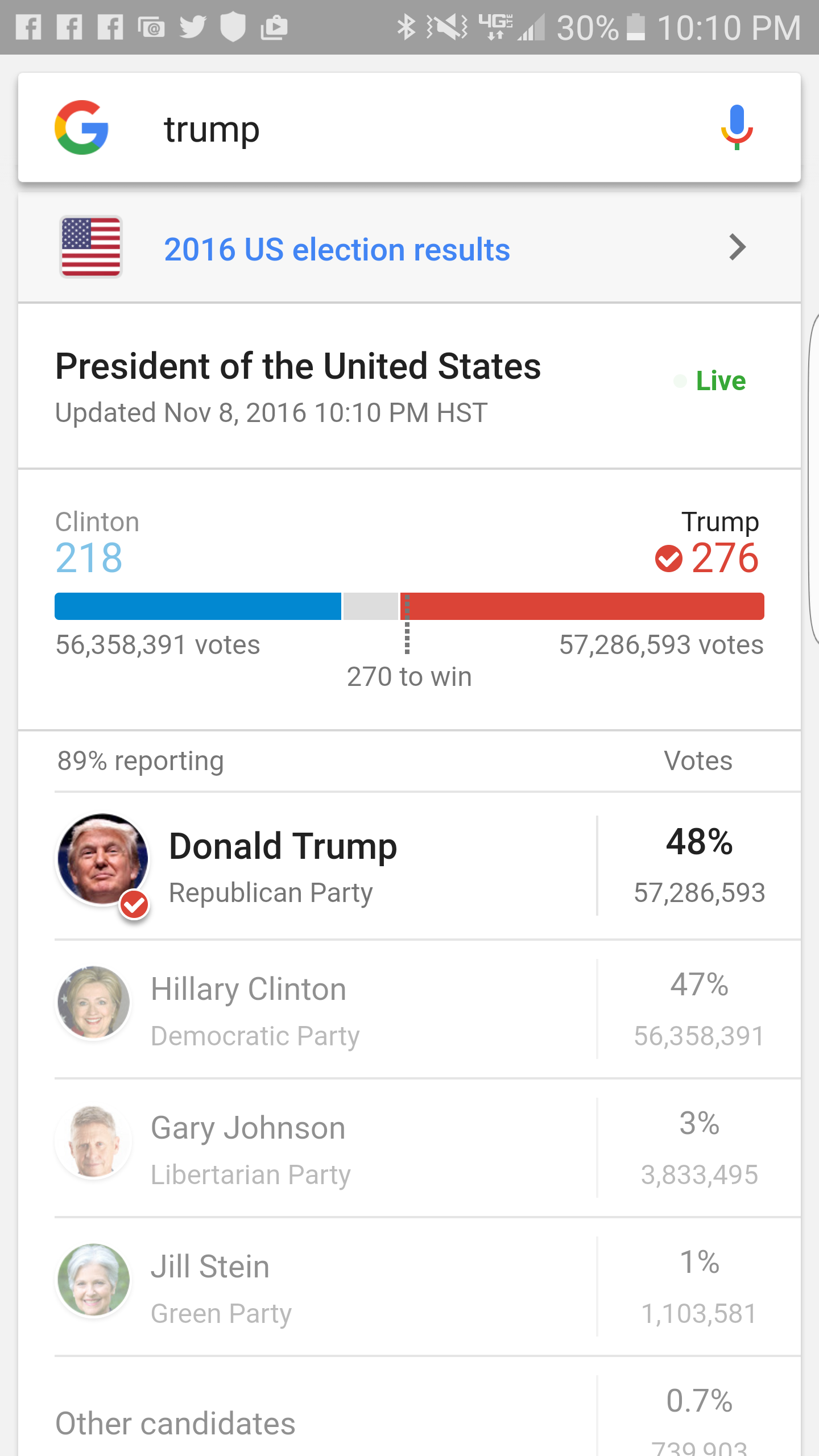This vertical screenshot depicts the 2016 U.S. election results as viewed on an Android phone at 10:10 p.m. with a battery level at 30%. The header features standard status icons, including time, battery, and three Facebook notifications on the left, as well as a Google search bar displaying "Trump" and a microphone icon beside the U.S. flag. Below this, in blue letters, are the words "2016 U.S. election results," followed by a green arrow pointing to the right and "President of the United States" in black text. The data is noted as updated on Nov 8, 2016, at 10:10 p.m. HST, with a "live" indication in green.

The election results are visually represented with green and red bars. Hillary Clinton's tally shows 218 electoral votes, while Donald Trump, designated by a red checkmark within a white circle, leads with 276 electoral votes. Clinton's popular vote count exceeds 56 million, while Trump's is over 57 million, with a note that 270 electoral votes are required to win. The results indicate 89% reporting at this time.

Further details include candidate profiles: Donald Trump, identified by his photo within a red check-marked circle, represents the Republican Party with 48% of the vote; below him is Hillary Clinton for the Democratic Party with her vote percentage displayed in gray. The Libertarian Party's Gary Johnson and the Green Party's Jill Stein follow, along with their respective vote percentages and other minor candidates.

This screenshot provides a snapshot of the real-time election night updates as they appeared on the viewer's phone, capturing the unfolding results of the 2016 U.S. presidential election.